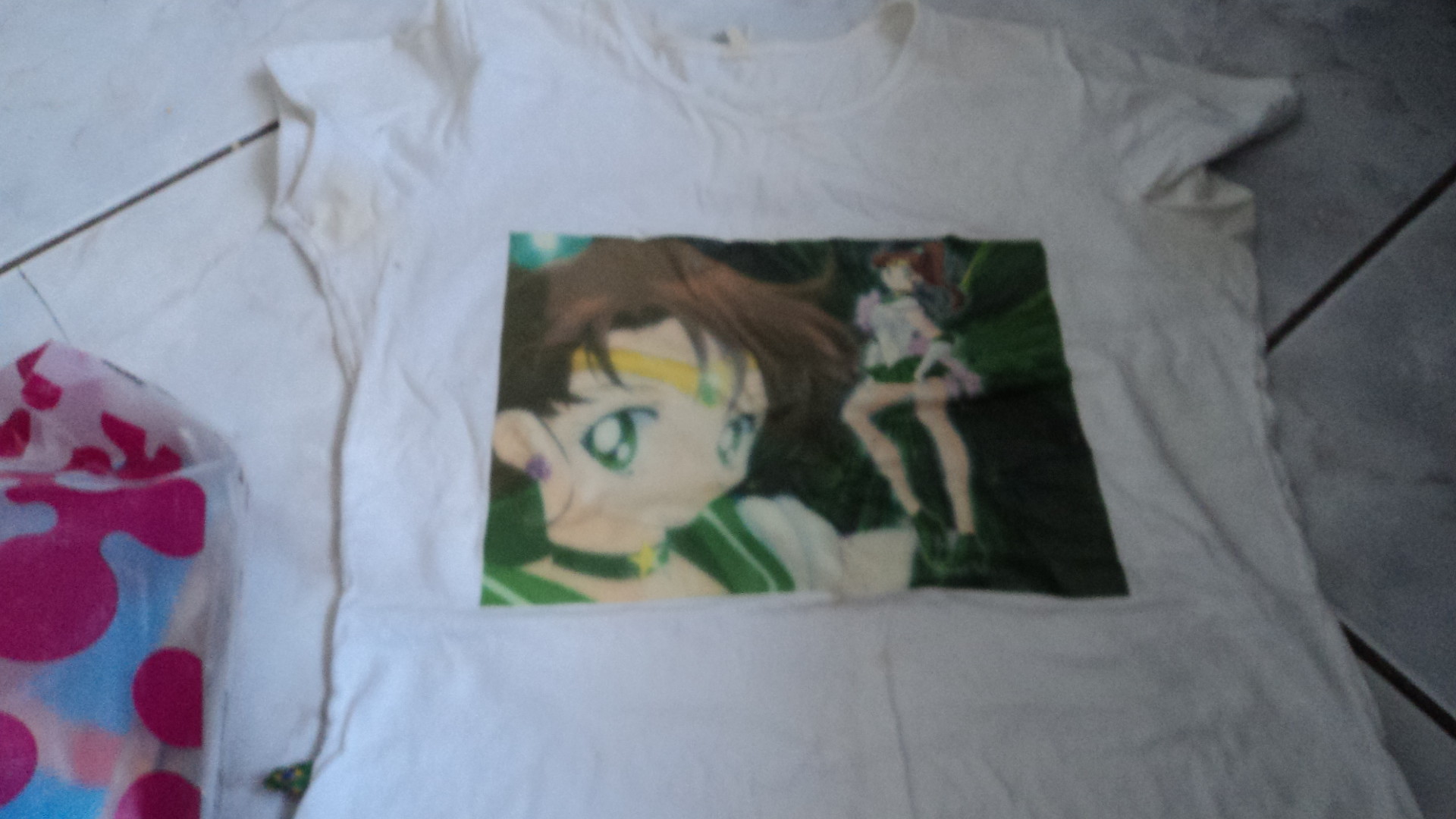This photograph captures a slightly angled, top-down view of a white tile floor with a fake marble-like finish and dark beige grout. Notably, the grout in the top left tile has a small missing spot revealing the white tile beneath. In the bottom left corner of the image, there is a clear plastic bag adorned with pink patterns resembling bubbles or splotches, with hints of a light blue object inside. Positioned to the right of the bag is a very wrinkled, short-sleeved white t-shirt with noticeable sweat stains under the arms. The shirt, which appears to be worn and slightly dirty, features an image of an anime girl with brown hair (possibly in a ponytail), green eyes, purple earrings, and a green choker with a star. The anime girl is depicted with short, swirling hair and large eyes, evoking a style reminiscent of Sailor Moon characters, although the exact character isn't entirely clear.